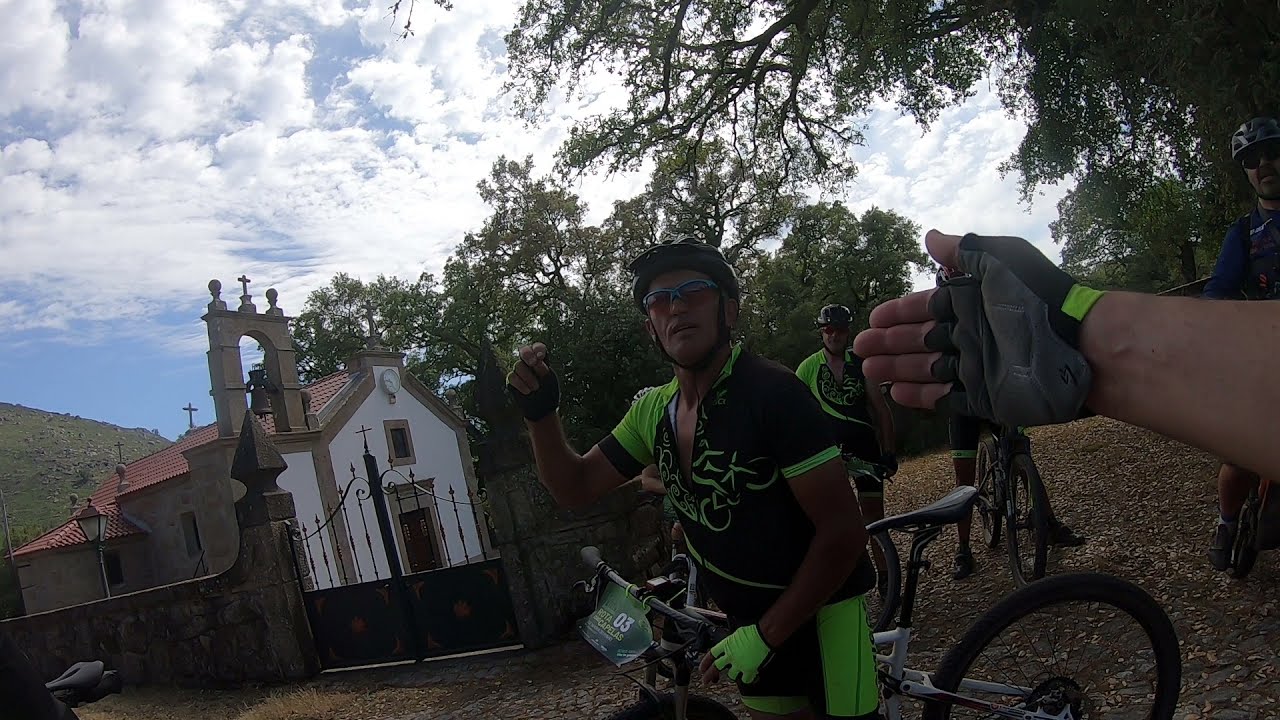In this point-of-view shot, the scene captures an outdoor cycling adventure featuring three individuals. The photographer's right hand, clad in fingerless gray, black, and yellow gloves, reaches out towards a cyclist who takes center stage in the image, wearing a black and lime green zippered shirt with short sleeves, matching tight shorts, and fingerless gloves. This cyclist also sports a black helmet and sunglasses; on the handlebars of their black and white bicycle hangs a banner displaying the number 03. Directly behind them rides another cyclist in an identical uniform and gear, including black helmets and glasses. The backdrop features a blend of natural and architectural elements: a cluster of trees, a sky partially filled with white clouds, and a small white church with a distinct red tiled roof and a cross atop a cement structure. The ground is scattered with leaves, and a gate leading to the church appears shut. The image exudes a sense of camaraderie and readiness for a biking excursion.